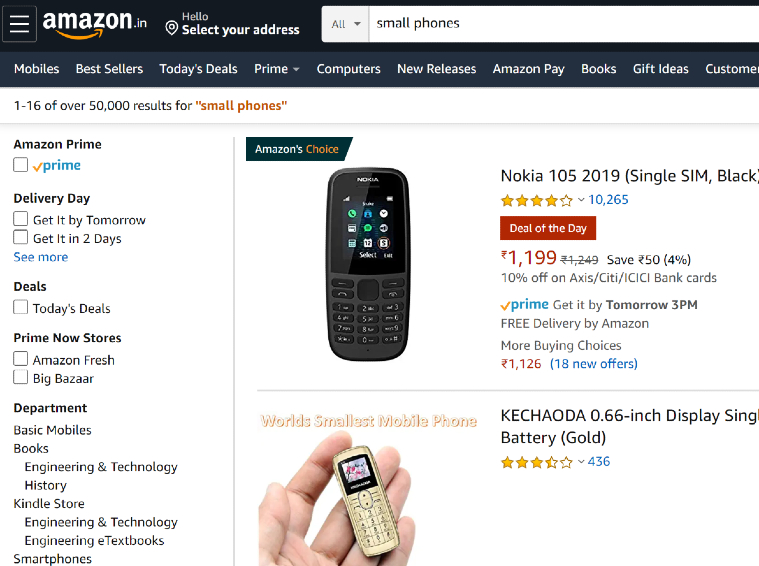This image is a wide-format screenshot of someone browsing Amazon, specifically shopping for a small phone. The screenshot captures two search results prominently. 

The first search result showcases Amazon's Choice: the Nokia 105, 2019 model, single SIM in black. It is listed as the 'Deal of the Day' priced at ₹1,199. The currency denomination is assumed to be Indian Rupees.

The second search result features the world's smallest mobile phone by the brand K-E-C-H-A-O-D-A. This phone boasts a 0.66-inch display and a gold-colored casing. Notably, this model from 2019 does not list a price in the screenshot.

This screenshot provides a glimpse into the online shopping experience on Amazon for compact mobile phones, highlighting specific details and options available to the user.